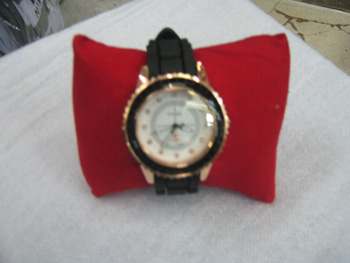This blurry photograph centers on a watch displayed prominently on a small red cushion, giving it the appearance of resting on a tiny pillow. The watch features a distinctive black band and a gold outer edge encircling the face. The watch face is primarily white, adorned with a black ring and what seem to be delicate hands that are difficult to discern due to the blurriness. Gold accents are interspersed along the band. The cushion and watch sit on a light-colored table, possibly light gray or white, with hints of tan in the background on either side, adding a subtle depth to the scene. The overall focus of the image is slightly compromised by its unclear quality, making finer details hard to make out.